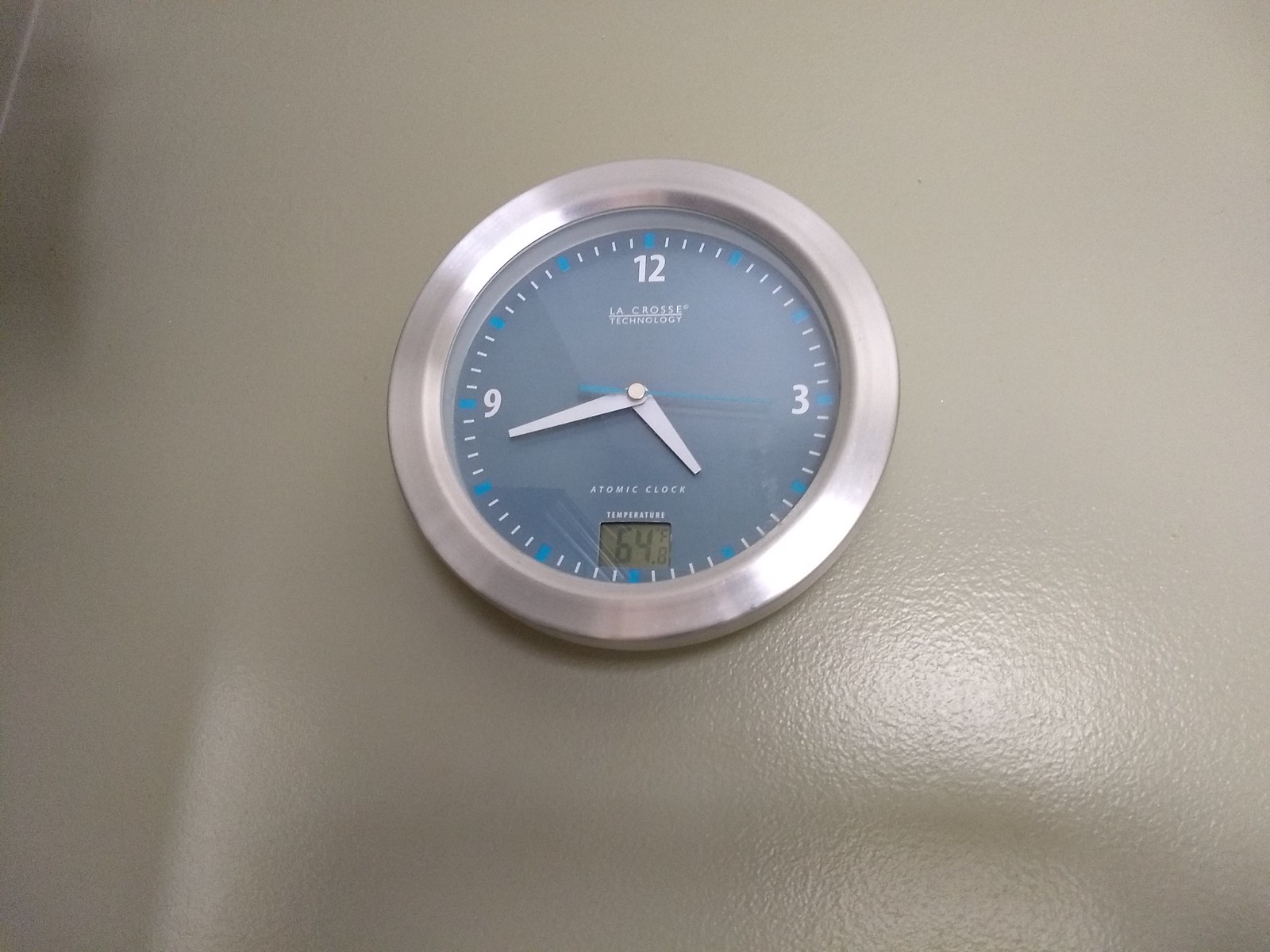This photograph captures a circular wall clock set against a light gray backdrop. The clock boasts a vibrant blue face encased in a thick, silver metallic rim that wraps around its top and sides. Prominently, the numbers 12, 3, and 9 are displayed in crisp white, while a small digital display replaces the numeral 6, exhibiting the digits "6" and "4" in black on a slightly off-white, almost dirty background. The clock's hands are robust and white, with the second hand standing out in a light blue hue. The hour markers are highlighted in a striking bright blue, while the minute indicators are presented in white to maintain clarity and balance within the design.